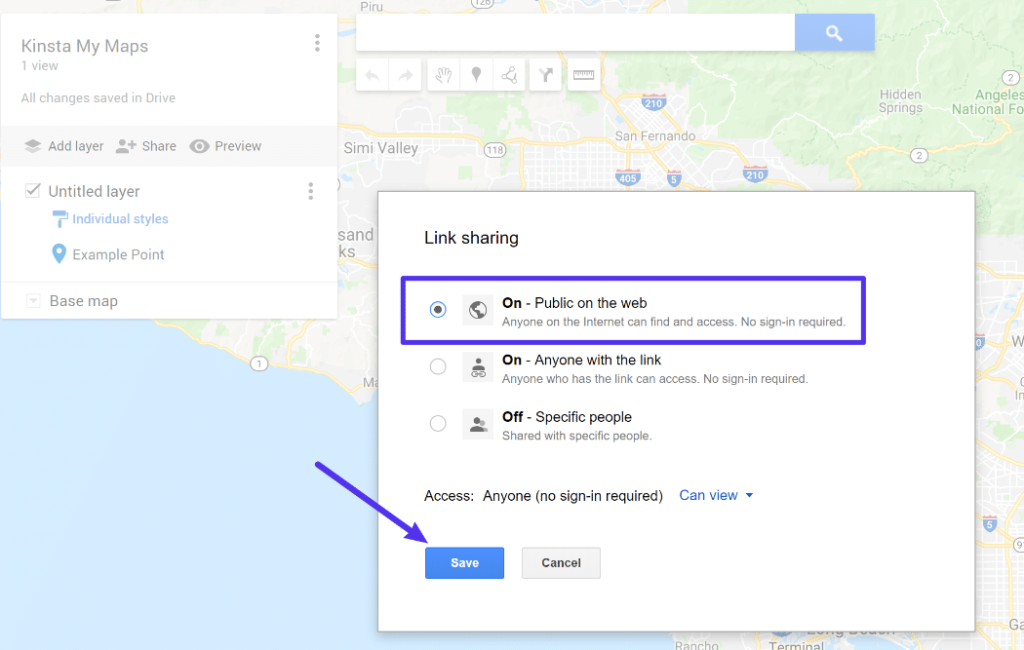The image depicts a digital map interface showcasing a detailed map of an area in California. The background features various colors: blue representing bodies of water, yellow for highways, and a mixture of gray and green for land areas. Prominent geographic names visible on the map are Simi Valley, San Fernando, Hidden Springs, and Angeles National Forest, suggesting the map covers parts of Southern California.

At the top of the interface, there is a white search bar accompanied by a blue search button. In the upper left-hand corner, a dropdown menu is visible, displaying options including "Kinsta," "My Maps," "One View," "All Changes," "Saved," "Drive," "Add Layer," "Share," and "Preview." An option labeled "Untitled layer" is checked, with additional settings for "Individual styles," "Example point," and "Base map."

A purple arrow points to a blue "Save" button located within a secondary pop-up window. This window details sharing settings, indicating that the map is publicly available on the web, with no sign-in required to access. The options listed include "Anyone with the link," "Anyone who has the link can access," and "Specific people." The selected access level is "Anyone on the web can view, no sign-in required."